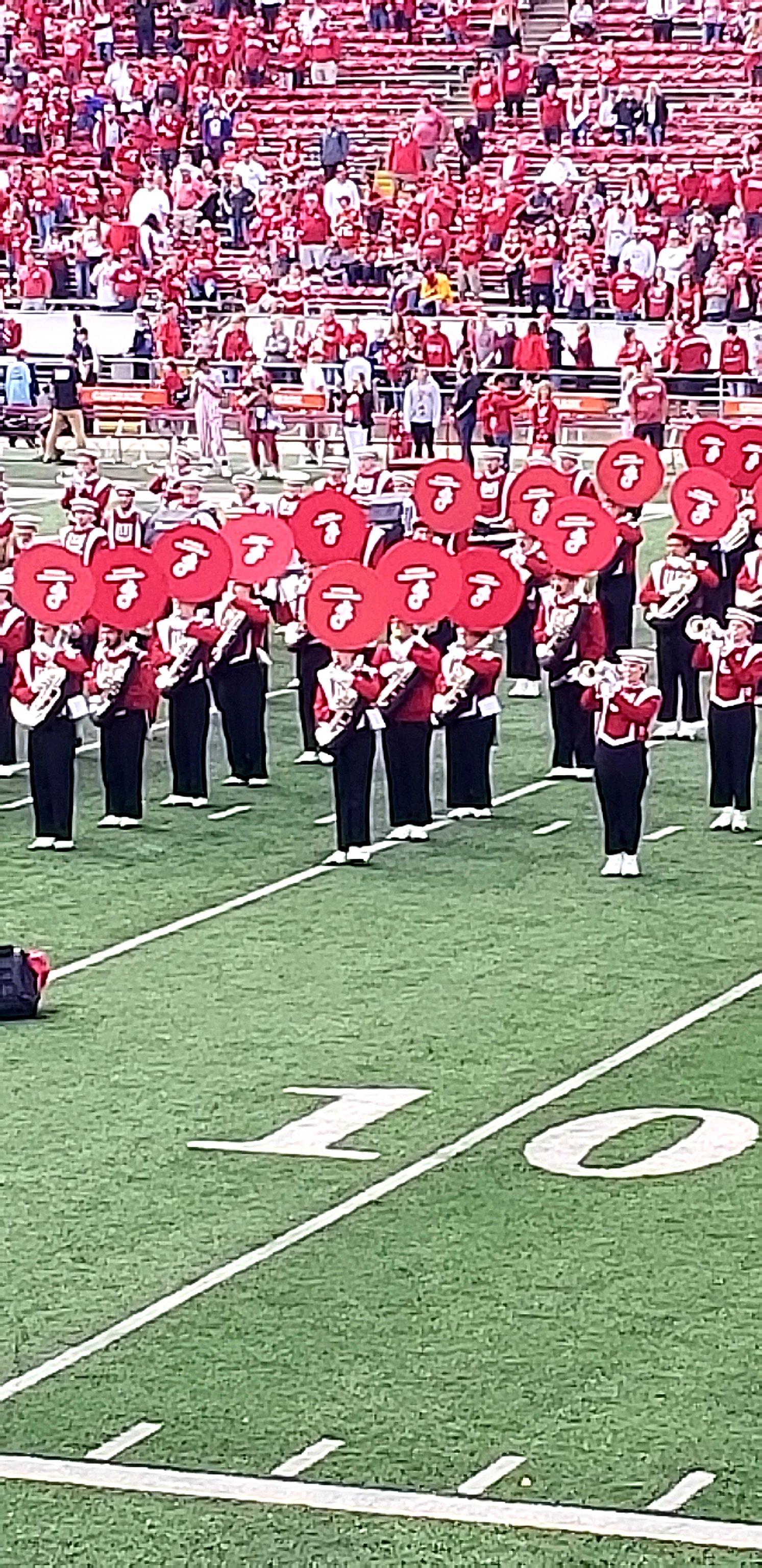The image captures a wide shot of a marching band performing on a football field, specifically positioned around the 10-yard line. All members are uniformly dressed in white shoes, black pants, red long-sleeve jackets with white trim, and short, flat white hats. The band includes various wind instruments, prominently featuring tubas with red covers bearing white logos. Nearby, a few trumpet players are visible. The stadium in the background is half-filled with attendees, most of whom are standing and dressed in red clothing, presumably supporting their team. The scene is lively, with a clear view of the field's 10-yard marker, sideline, and the red-seated grandstands extending upward.